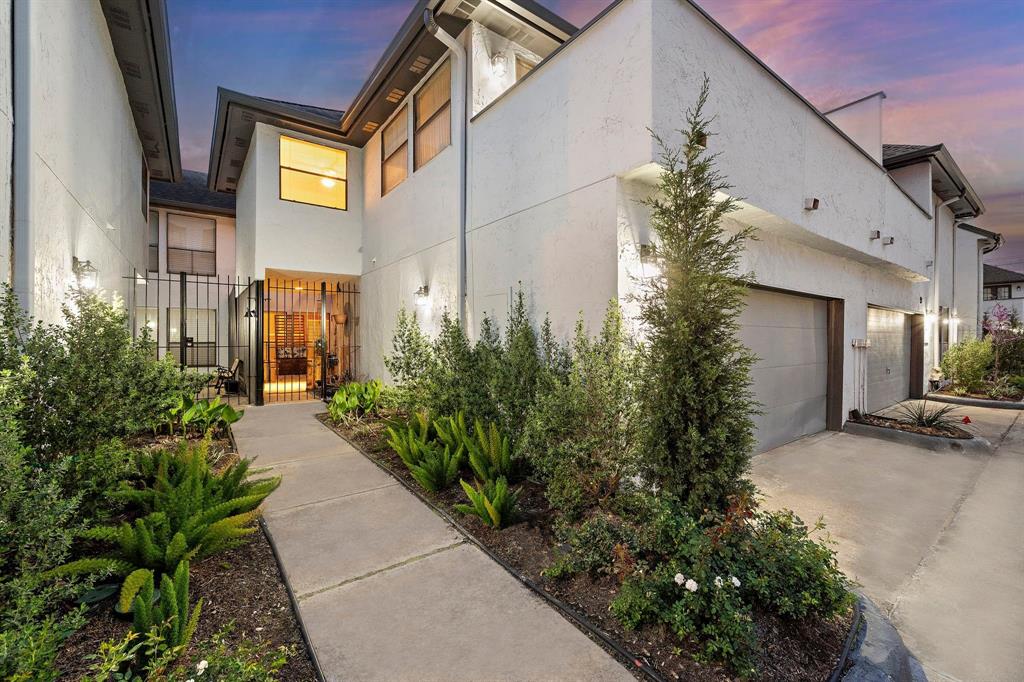The image showcases a contemporary row of townhouses or condos built in a modern, boxy style and featuring white stucco siding. These two-story structures have dark, slightly pitched roofs, and the overall aesthetic is clean and minimalist. Each unit has a grayish metal garage door at the front, with strategically placed lights illuminating the area. The driveway slabs and adjacent concrete sidewalks are neatly laid out, leading to a central wrought iron gate that adds a touch of gothic elegance. The gate opens to a concrete walkway flanked by a variety of plants, shrubs, flowers, and small trees, emphasizing the well-maintained greenery between the garages and along the path. The scene appears to be taken during dusk, as there is a darkish blue and purple sky with some clouds, with lights on inside and outside the house, adding a warm glow to the modern architectural elements. The top-floor balconies, sitting above the garages, further contribute to the contemporary look of the townhouses.